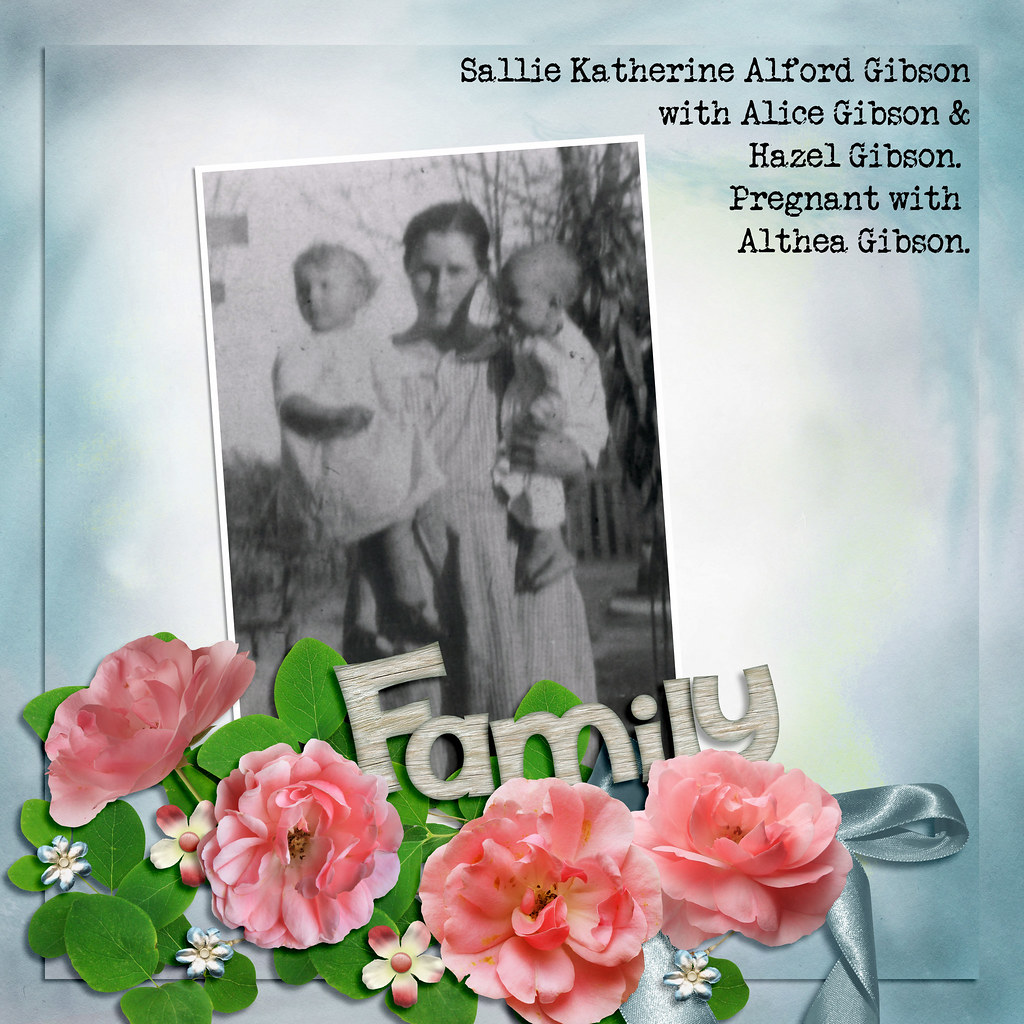The image is a meticulously crafted blend of vintage photography and vibrant graphic design, resembling the front cover of a family photo album. Central to the composition is a black-and-white photograph of a woman standing in a yard, holding two small children—one in each arm—with trees visible in the background. Beneath the photograph, towards the bottom of the image, are realistic-looking pink roses accompanied by green leaves and a blue ribbon. The word "Family" appears in a prominent white font over the floral arrangement. The background of the image features a soft, light blue square, adding depth and creating the effect of layered paper. In the upper-right corner, black typewriter-style text reads: "Sally Catherine Alfred Gibson with Alice Gibson and Hazel Gibson pregnant with Althea Gibson," providing context to the historical moment captured in the photograph. The overall color palette includes hues of pink, green, light blue, white, yellow, blue, and varying shades of gray, enhancing the visual appeal and nostalgic atmosphere.